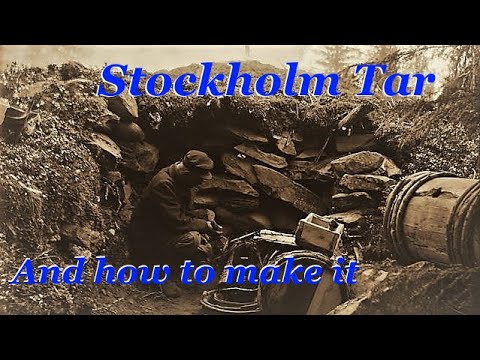The image appears to be a monochrome, movie-like frame featuring a man seated in a natural setting, possibly initiating a slideshow or presentation. The top and bottom of the image are bordered by black rectangles, overlaid with bold blue text outlined in white. At the top, it reads "Stockholm Tar," and at the bottom, it says "How to Make It." The man, wearing a darker jacket and a hat, is engaged in an activity with his hands, though the exact task is unclear. He is positioned near a stone wall, accompanied by several wooden barrels and a wooden box. Behind him is a dirt hill, and the scene is scattered with rocks, enhancing the rugged, outdoor atmosphere.